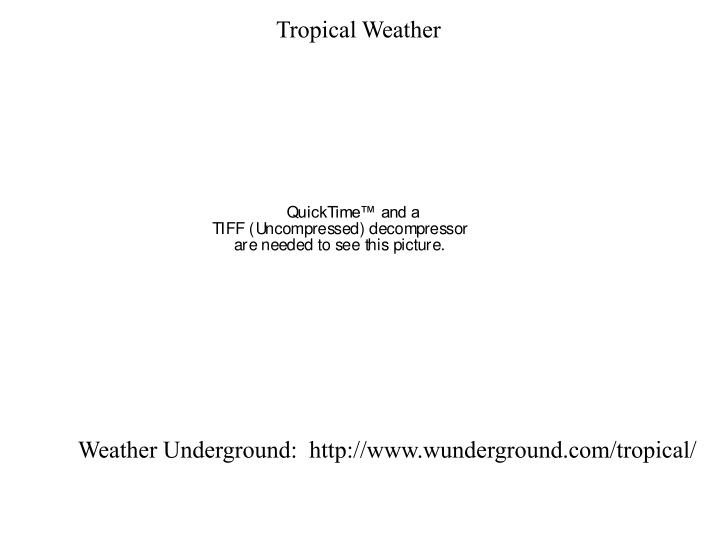The image consists of solely text in black (or dark gray) on a white background. At the top, the text reads "Tropical Weather," with both 'T' and 'W' capitalized. Below there is a noticeable space, followed by a paragraph that states: "QuickTime™ and a TIFF (Uncompressed) decompressor are needed to see this picture." The 'TM' symbol is positioned in the upper right corner of 'QuickTime'. At the bottom of the image, another space separates the paragraph from the final line of text, which reads "Weather Underground: http://www.wunderground.com/tropical/". The text appears as if it is from a webpage, with all elements presented in a horizontal and square orientation.